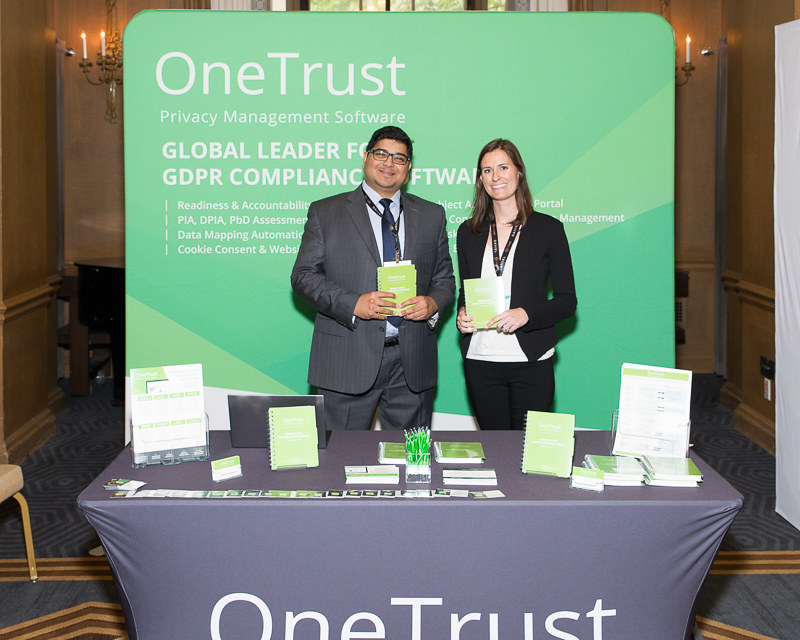This is a color photograph of a man and a woman standing at a display booth, likely at a trade show. They are positioned in front of a large green sign that prominently features the text "OneTrust" in white. Below the main text, additional text reads "Privacy Management Software, Global Leader," though some of the details are obscured by their presence.

The man is dressed in a grey suit paired with a white shirt and blue tie. He has black hair, wears glasses, and appears to have an Asian complexion. The woman beside him has brown hair and is wearing a white T-shirt under a black jacket, complemented by black pants.

In front of them is a table covered with a blue tablecloth that also displays the "OneTrust" branding. The table is cluttered with various promotional materials, including pamphlets, business cards, and a noticeable cluster of green pencils. The photograph also captures the ambiance with its beige walls adorned with illuminated wall sconces and a multicolored carpet visible at the bottom edges.

Overall, the image effectively depicts a professional and informative setup, representing OneTrust at a trade show event.